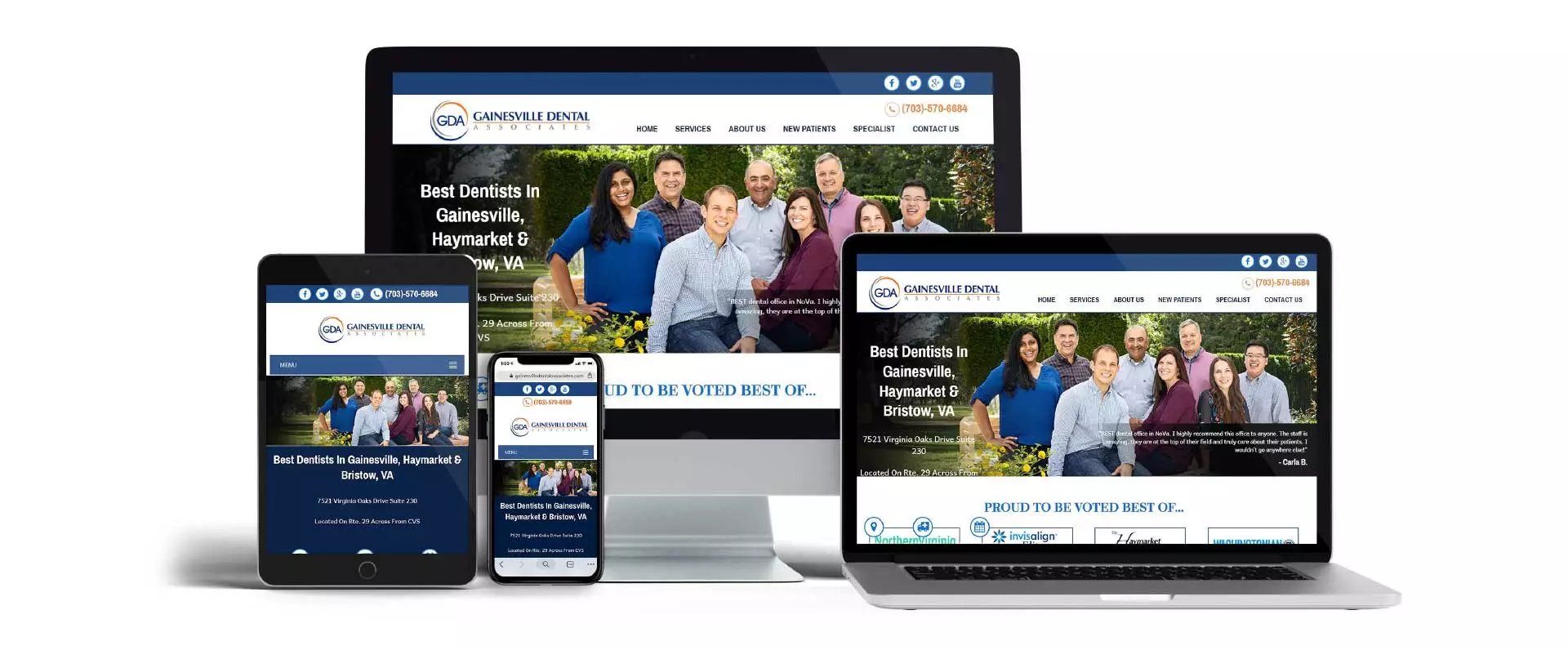This image, predominantly white with no distinct boundaries, captures a series of technological devices arrayed neatly side by side, all displaying the same dental website. Positioned slightly left of center is a standard computer monitor, presented in widescreen with a silver base and black bezel. Dominating its screen is a webpage highlighting a dental office, proclaiming "Best Dentist in Gainesville," with an accompanying photograph of the office staff.

Below this monitor and to the lower left sits a tablet, its display also showcasing the same dental website. To the immediate right of the tablet, a smartphone stands upright in a vertical orientation, mirroring the web page to maintain consistency. Completing the ensemble is a laptop on the lower right, its screen too synchronized with the others, reinforcing the uniformity of the content presented.

The concise alignment and uniformity of the devices emphasize the informative dental page, creating a cohesive visual narrative focused on the technology and the shared digital content.